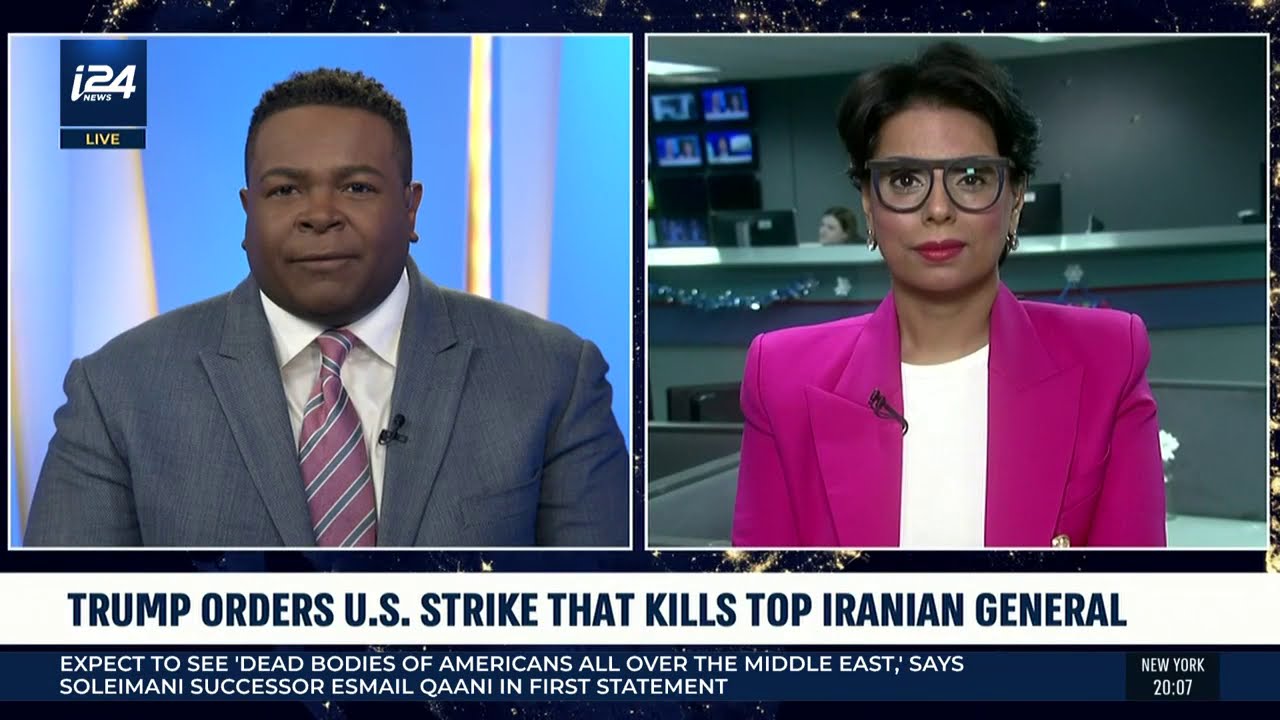The screenshot from a TV news broadcast displays two individuals in separate square blocks against different backgrounds. On the left is a heavily built African American man with short, slightly curly black hair. He is wearing a light gray suit jacket, a white collared button-up shirt, and a pink tie adorned with blue vertical stripes. A lapel microphone is clipped to his jacket, and the overlay text "I24 News Live" is visible at the top left corner of his screen. The woman on the right, who has brown skin and short dark brown hair, is wearing a pair of thick-framed glasses with a flat brow rim. Her outfit includes a fuchsia lapel jacket over a white shirt, complemented by a lapel microphone. The background features a counter, a lady, some news screens, and cubicles. Both anchors are looking straight at the camera with neutral expressions. At the bottom of the image, a white banner with blue writing states, "Trump orders US strike that kills top Iranian general," followed by a blue banner with white writing that declares, "Expect to see dead bodies of Americans all over the Middle East, says Soleimani successor Esmail Khani in first statement." The timestamp "New York 20:07" appears in a small black box with white writing on the lower right.